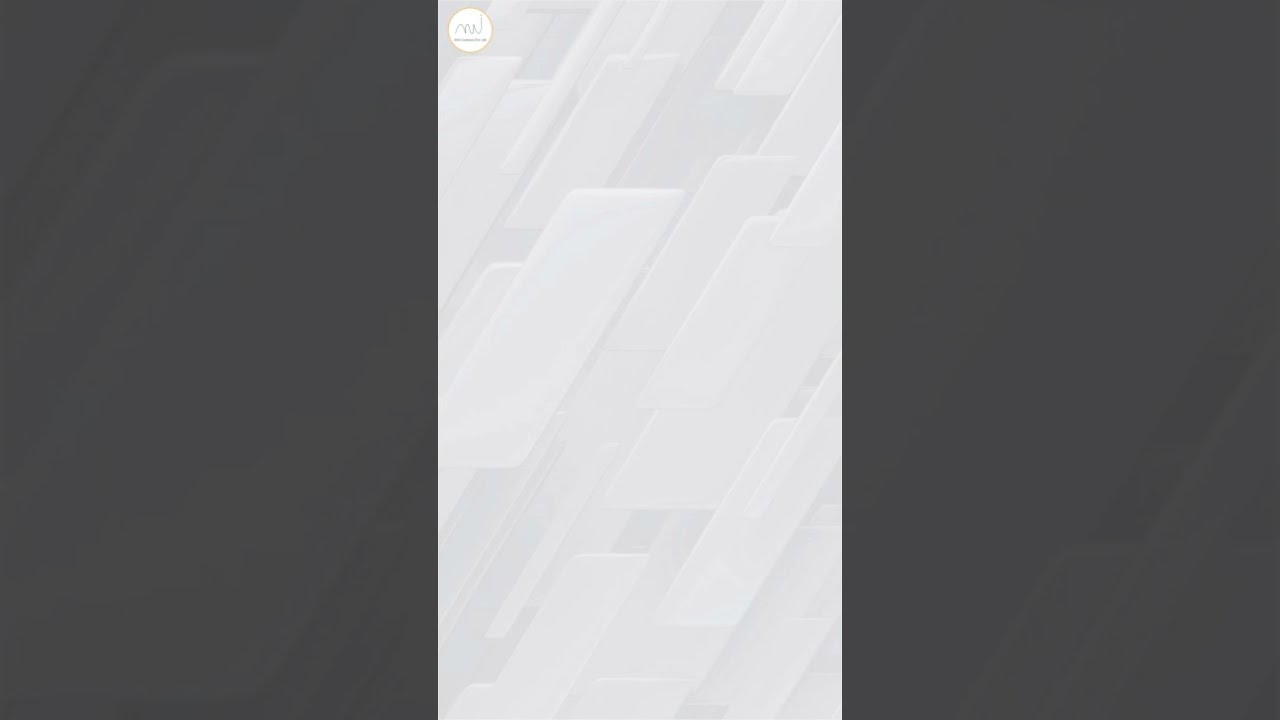The image is a rectangular, abstract composition divided into three sections. The central section is a light gray rectangle, featuring diagonally slanted planks that resemble a hardwood floor pattern, transitioning from the bottom left to the top right. These planks vary subtly in shade, adding a sense of texture and dimension. At the top left corner of this gray segment, there's a small white circle with a hint of yellow and some indistinguishable, squiggly writing. On either side of this central section, there are darker, zoomed-in rectangular portions of the same plank pattern. These side sections are in deep gray tones, making the outlines of the hardwood-like planks appear obscured but still discernible. The entire composition evokes a stark, almost flag-like appearance, with its contrasting light and dark elements and the intricate, textured details in the center.